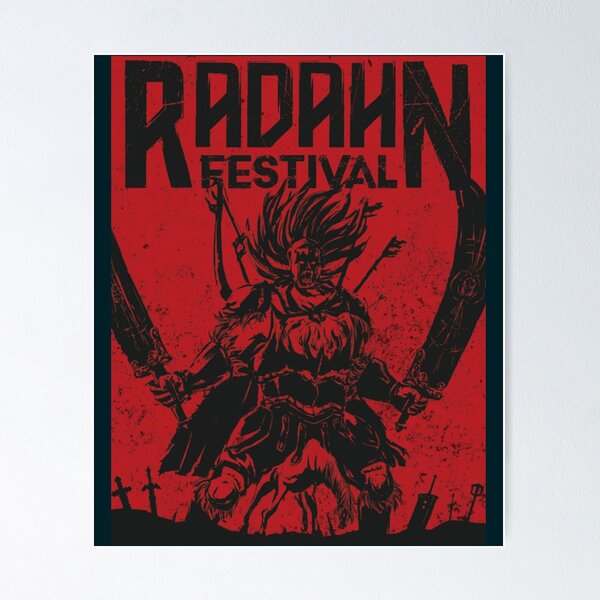This square-oriented festival poster boasts a dark deep red background bordered by a thick light gray frame. The top of the poster prominently features the name "RADAHN" in bold black letters, with an oversized R and N flanking the smaller letters A-D-A-H. Nested between the R and the N is the word "FESTIVAL," also in black capital letters. Dominating the center of the poster is an imposing figure—predominantly drawn in black—that appears to be a demon warrior. This menacing character faces forward with wild, flame-like hair shooting upward and a headdress resembling black flames. His powerful arms stretch out with elbows bent, gripping large, intricately etched weapons or banners in both hands. His burly frame is clad in heavy armor, adorned with fur and various accouterments. The ground below him is punctuated with an assortment of items, including knives and swords embedded in the earth, with a partially obscured shape between his legs that vaguely resembles a horse. The overall imagery exudes a sense of dark, feral power, encapsulating the fierce and chaotic spirit of the RADAHN festival.